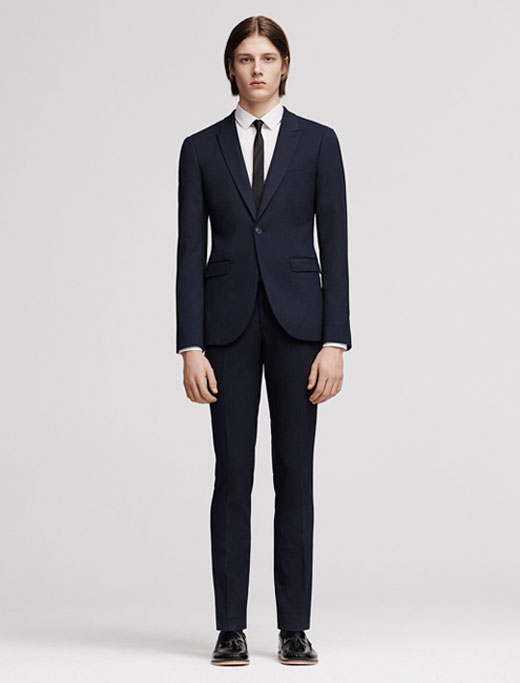In the image, a tall, thin man with a somber expression stands in the center, modeling business attire against a light gray or grayish white background. He has pale skin and blue eyes, giving him a distinctly Caucasian appearance. His neck-length hair is parted in the middle and falls neatly to both sides. The man is wearing a dark blue suit with a single button and two pockets on either side. Underneath, he sports a white collared shirt paired with a thin black tie. His attire is completed by shiny black leather shoes, which feature tan soles. The man's hands hang unnaturally at his sides, emphasizing the serious and slightly bored expression on his face. His overall look is androgynous, and his large hands contribute to the slightly awkward stance.